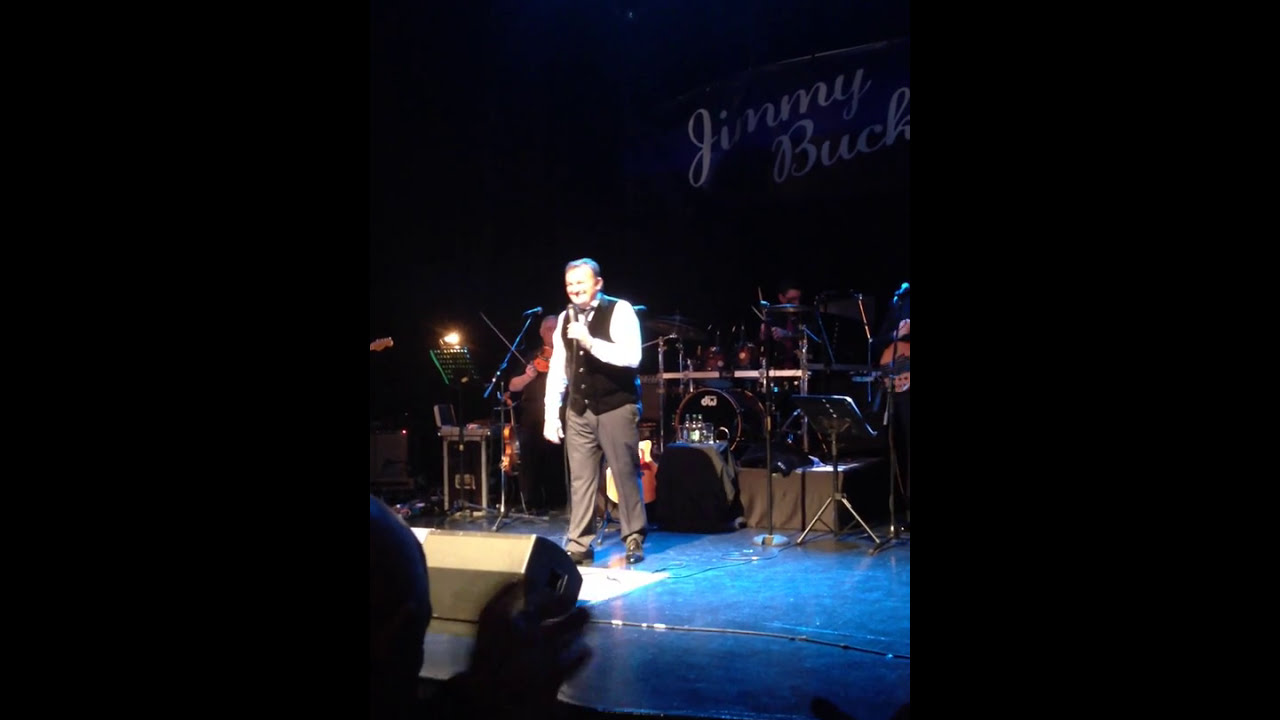The image captures a lively stage performance featuring a middle-aged man at the forefront, dressed in a black vest over a white long-sleeve shirt, and gray dress pants with crease lines. He is smiling and holding a microphone to his mouth. Behind him, a vibrant setting unfolds with a drummer playing on a predominantly red and black drum kit. The drummer is partially obscured but identifiable, with cymbals and drumsticks clearly visible. To the man's left, partially hidden, are musicians including a person holding a violin or cello and another holding a guitar. Mic stands, metal stands for sheet music, and an acoustic guitar set up nearby add to the scene's musical ambiance. The stage is distinctly marked by a bright royal blue floor, and prominently above the performers, the name "Jimmy Buck" is displayed in large, cursive white letters. Additionally, there are small details like a black-clothed table with drinks. In the lower left corner, a single silhouetted figure in the audience can be seen, contributing to the atmosphere of a live performance, with the rest of the audience obscured in the darkness of the background. The overall scene is well-lit, with a spotlight on the central performer, suggesting the image was likely taken on a cell phone, as indicated by the vertical cropping and black bars on either side.